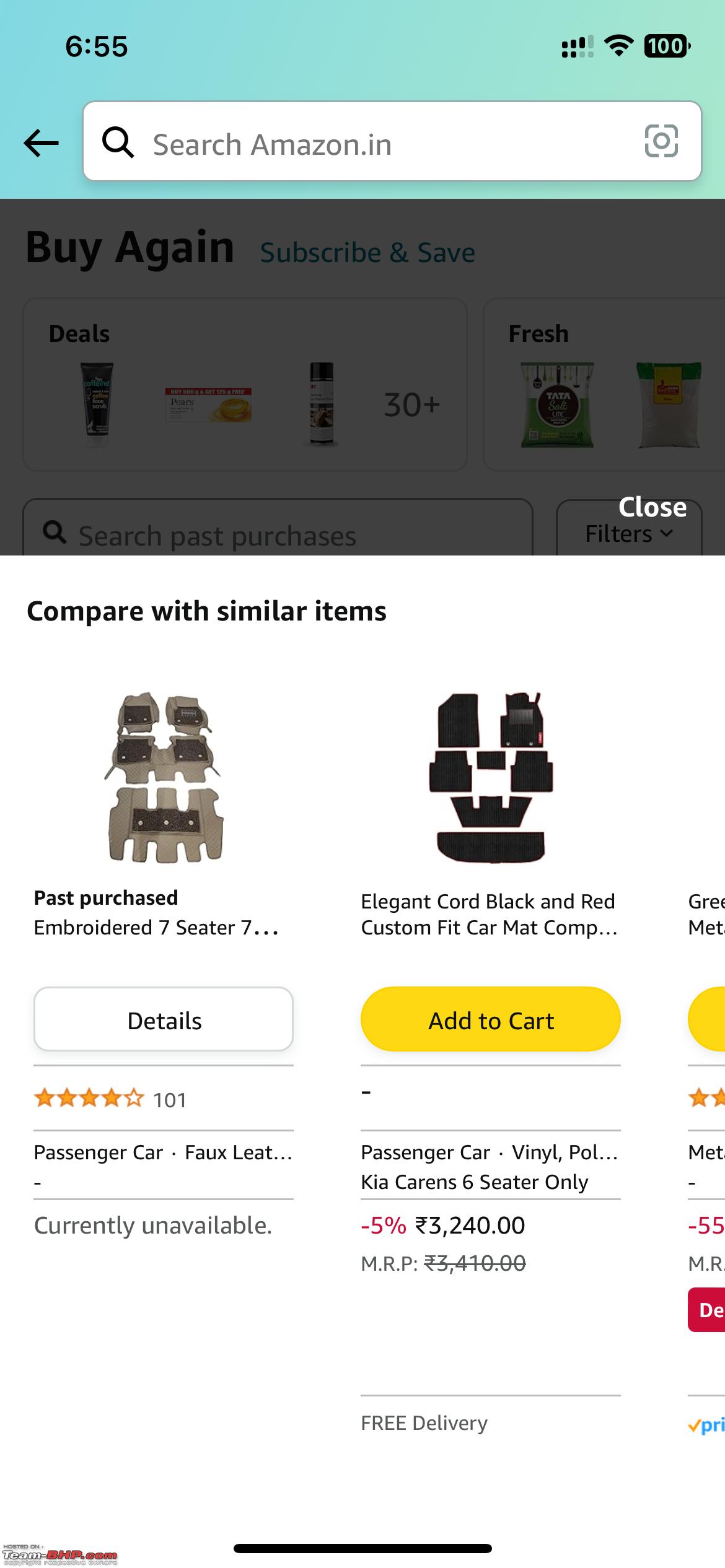The image depicts the Amazon app interface on a smartphone screen. At the top of the screen, the device status indicators show the time as 6:55, a full Wi-Fi signal, and a 100% battery level. Below the indicators, a prominent search bar reads "Search Amazon.in," accompanied by a black magnifying glass icon and a camera icon for visual search options. To the left of the search bar is a back arrow, and the overall color scheme features light blue and green hues.

The main content of the page includes a pop-up window with the heading "Compare with similar items." The first item listed is a previously purchased "Embroidered Seven Seater," which boasts a four-star rating and 101 reviews but is currently unavailable. Categories tagged under this item include "Passenger Car."

The second item showcased is an "Elegant Cord Black and Red Custom Fit Car Mat," also categorized under "Passenger Car" and specified for a "Vinyl Kia Currents Six Seater Only." This product is black in color, offered at a 5% discount with a striking yellow "Add to Cart" button, priced at $3,240 (currency unspecified), and includes an option for free delivery.

Surrounding the pop-up are other features typical of the Amazon app, such as sections titled "Buy Again," "Deals," and "Fresh," along with another search box specifically for past purchases.

Overall, the detailed layout and features clearly indicate the familiar interface of the Amazon app commonly used on smartphones.